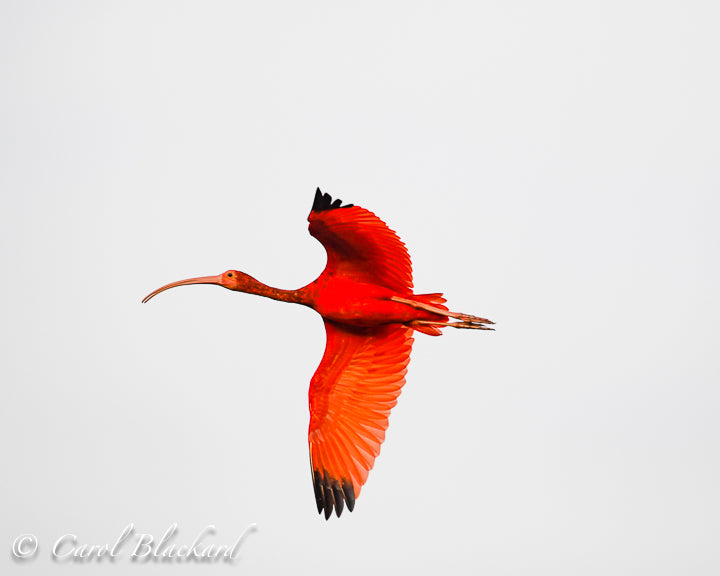This photograph captures a side view of a vibrant bird in flight, prominently displaying its strikingly red plumage. The bird features wings that span wide, showcasing a gradient of colors including orange hues near the wing base and black tips. Additionally, minute black or dark red spots adorn its neck. The bird's face carries an orange tint, and it possesses a long, slightly downward-curved beak, pink in hue. Its legs are tucked gracefully behind as it soars against a light gray sky. In the bottom left corner, the image is credited in elegant, white cursive text with a light drop shadow, reading "© Carol Blackard."